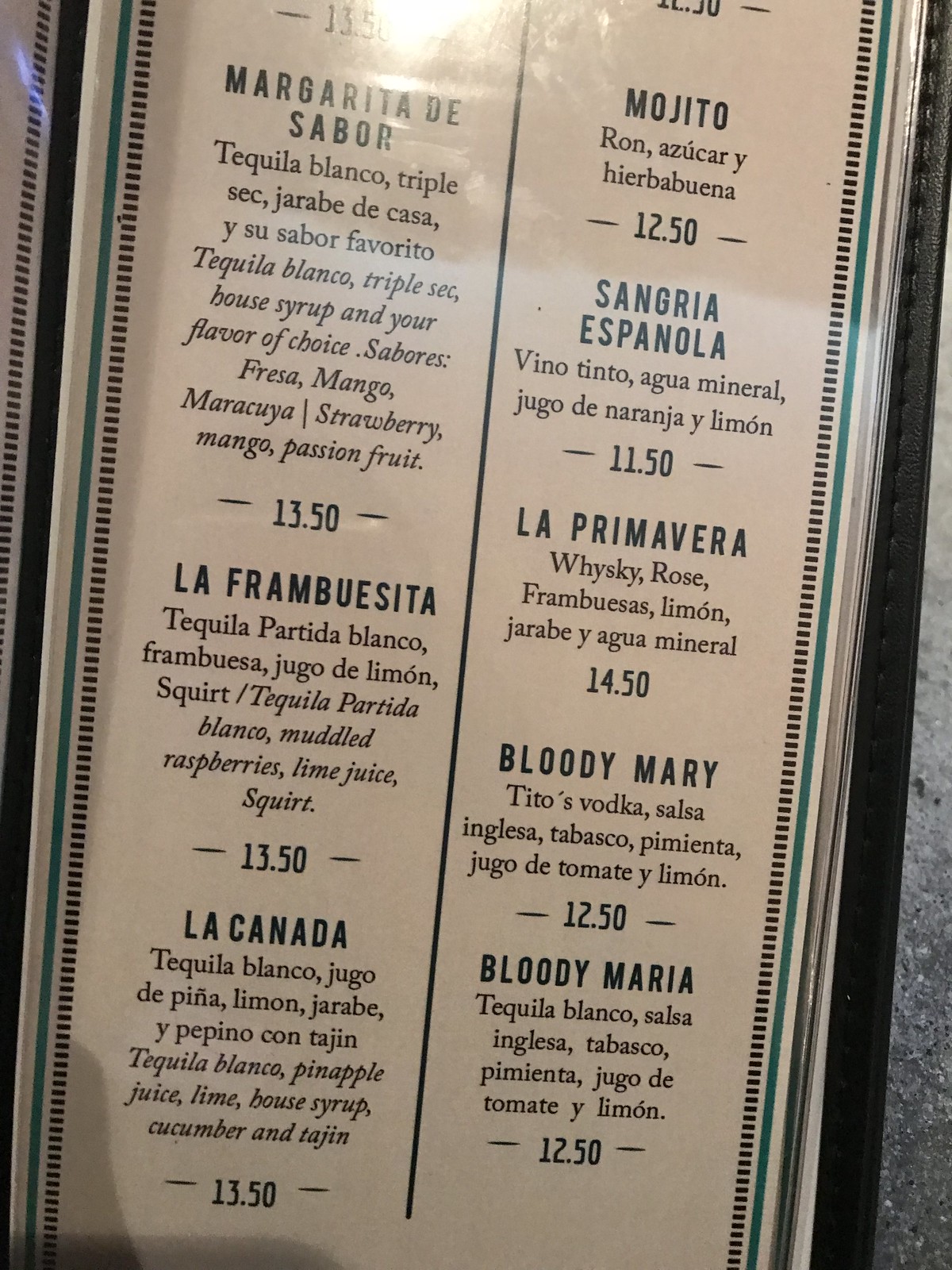This image features a streamlined drink menu encased in an elegant leather holder. The menu is organized neatly with a black font against a simple backdrop, highlighted by a green trim that borders the edges and a central divider. Each drink listed is priced uniformly at $13.50. The selection includes seven options: Margarita Sabor, Frambrocetta, La Cañada, Mojito, Sangria, La Primavera, Bloody Mary, and Bloody Maria. The layout is accessible and visually appealing, emphasizing the concise but varied offerings of refreshing beverages.